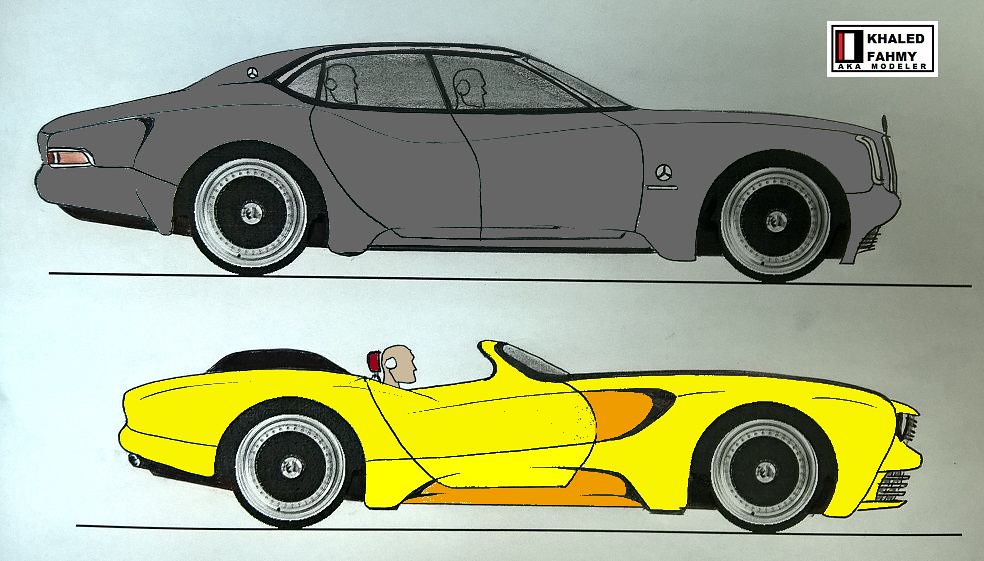This graphic illustration is divided into two segments, each featuring a side profile of a different car. The upper half displays a gray, four-door car with outlined silhouettes of a person seated in the front seat and another in the back seat, highlighting its family-oriented design. In contrast, the lower half showcases a vibrant yellow, two-door sports car with the outline of a solo driver, emphasizing its sleek and sporty appearance. A white box located in the top right corner contains the text "Caled Family, a.k.a. Modeler," suggesting a comparison or promotional context for these vehicles.